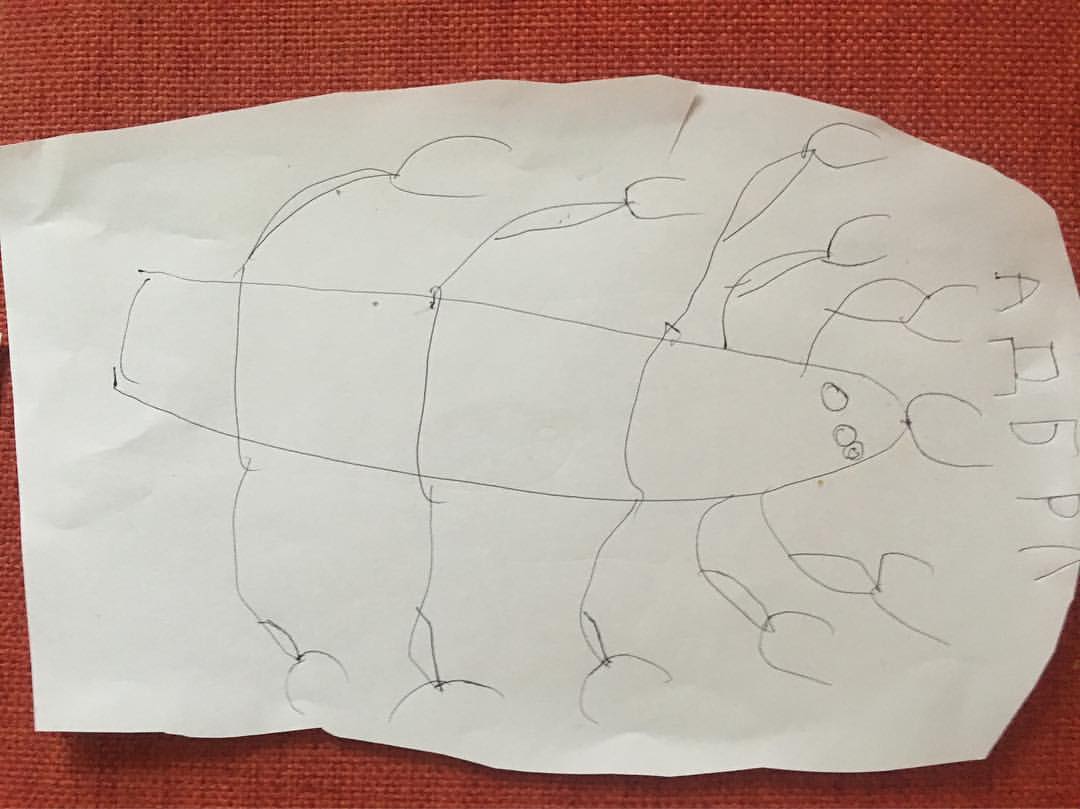This photograph showcases a meticulously drawn illustration on a cut-out piece of white paper, prominently placed against a red fabric backdrop. The artwork depicts a detailed lobster-like creature, oriented towards the right side of the image. It features at least ten legs and distinctive pincers at the top, along with three eyes positioned near its head. Above the lobster, there are five Cyrillic letters, with discernible characters resembling "A", "P", and another "A" without the horizontal bar, though the other letters are unclear.

The drawing appears to be rendered in pencil or a fine black ballpoint pen, demonstrating intricate line work and shading. Dominating almost the entire frame, the cut-out cast dark gray shadows on the red fabric, adding depth to the composition. The photograph is well-lit, likely taken either during the day or in a brightly-lit indoor setting, as evidenced by the even illumination and absence of pronounced light sources.